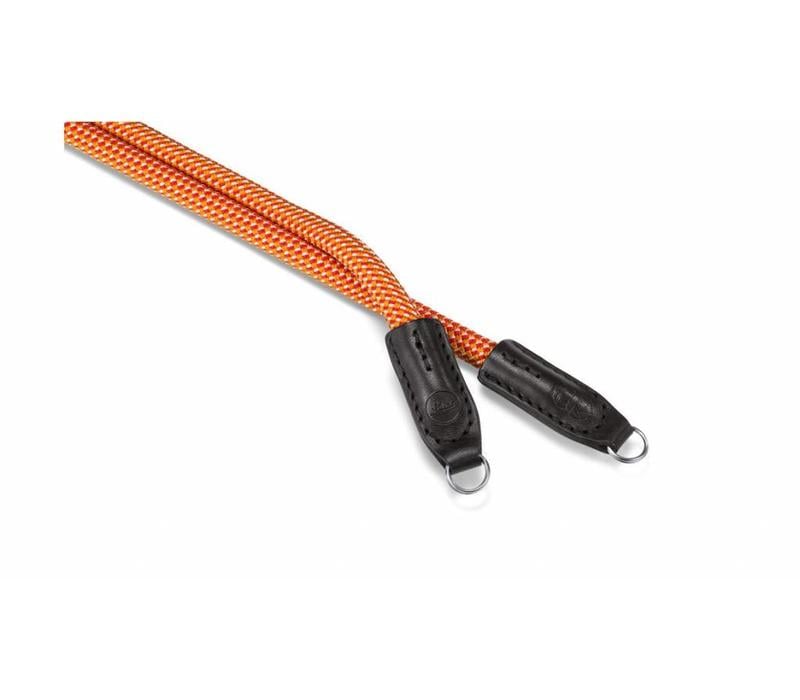The image features a skipping rope placed on a white surface, where only part of the rope is visible. The skipping rope comprises two black leather handles, each adorned with a logo and patterned design, including multiple small pinholes that give a curved flair. The ends of the handles have silver metal rings attached. The rope itself is thick and tightly woven into a checkerboard pattern of tan, orange, and red squares. The handles measure approximately two to three inches, and they cross over each other, with one handle neatly laid across the other.